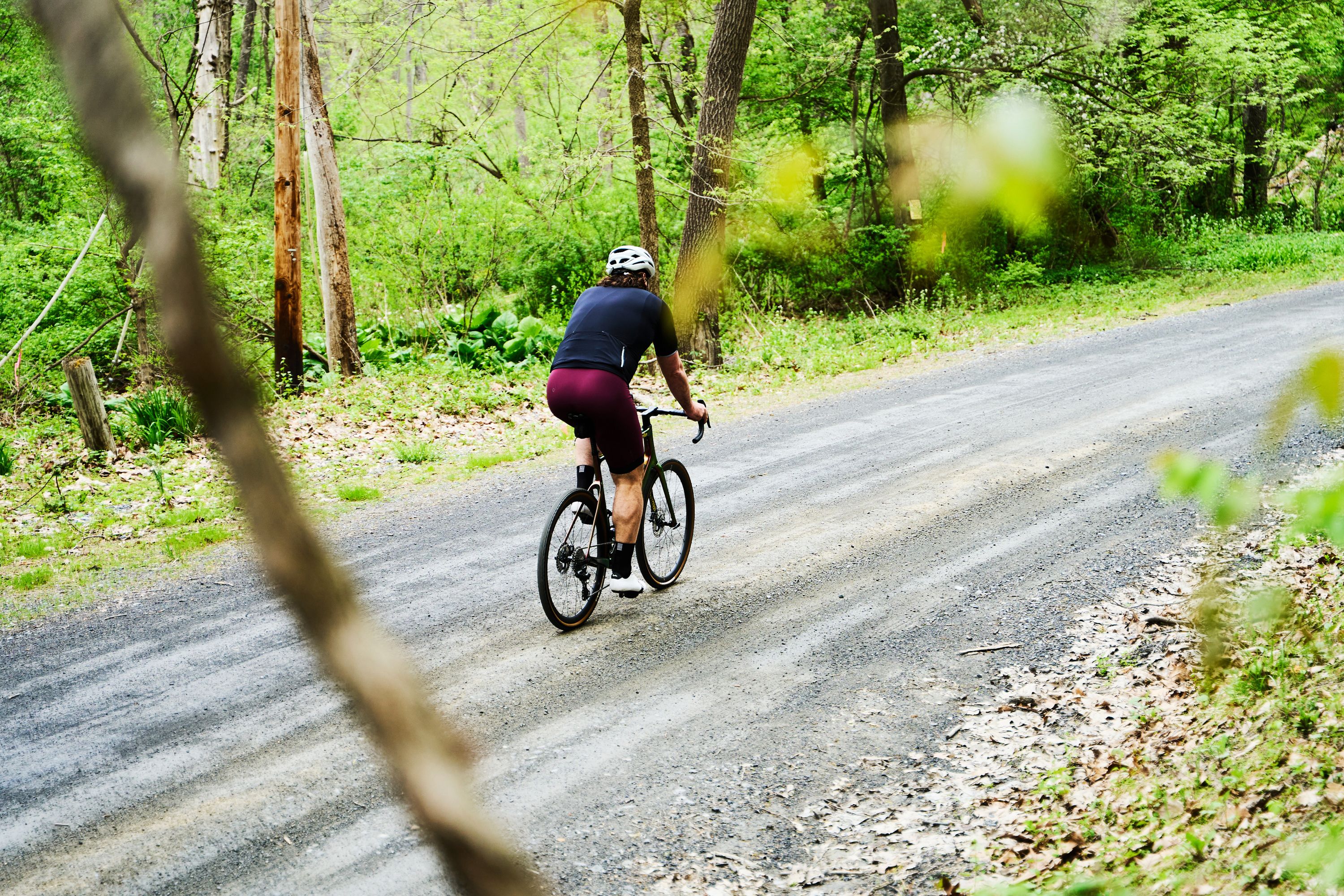In the foreground of the image, through a partially obscuring tree branch and some blurry leaves, the back of a bicyclist can be seen riding away on a gravel road. The cyclist, a man with muscular calves, is wearing a blue short-sleeved shirt, burgundy (almost purple) bicycle shorts, black socks, and white shoes. A white helmet sits atop their head. They are bent over the handlebars of their black mountain bike, which is leaning forward as if in a speed posture. The road they are on is lined with tall trees and dense forest, with bushes and brown, dead leaves scattered on either side. The lush greenery in the distance contrasts with the earthy tones surrounding the path. The setting appears to be a forest trail on a cloudy day, adding a serene yet dynamic atmosphere to the scene.